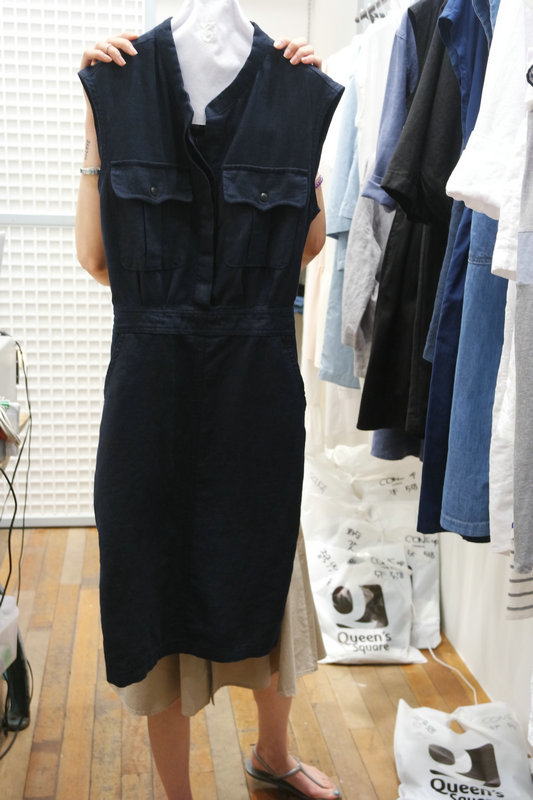In the photo, a woman is standing inside what appears to be a dressing room, holding up a large sleeveless black dress on a hanger in front of her, obscuring her face. The black dress reaches just below the knees, has pockets on the left and right breast, and features a low-cut neckline with a cinched waist. The woman is dressed in a light tan, almost cream-colored dress and is wearing sandals with her toenails painted a blue color. She stands on wooden floorboards, and surrounding her is a detailed scene: to her right, several dresses in white, blue, and black hues hang on racks, and below them are white bags with a black square logo and a white Q, labeled "Queen's Square". To her left, some wires dangle from an unidentified electronic device. In the background, there is a white checkered pattern and a white door can be seen behind her.